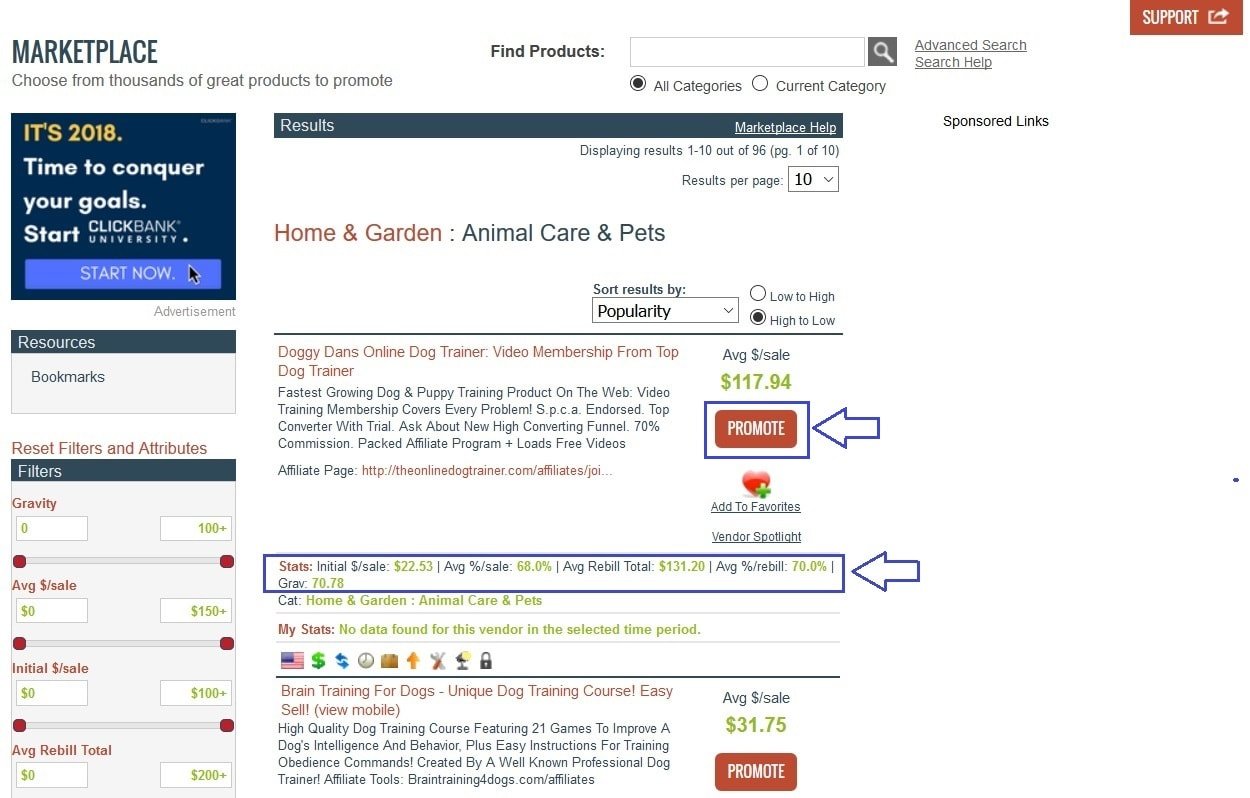The image depicts a promotional banner for an e-commerce or affiliate marketing platform, likely ClickBank, renowned for its affiliate marketing opportunities. The top of the image displays a header reading "Marketplace - Choose from Thousands of Great Products to Promote," clearly indicating the website's purpose. Beneath this, a motivational tagline reads, "2018: Time to Conquer Your Goals. Start ClickBank University. Start now." This suggests that the banner is from the year 2018 and encourages users to join ClickBank University to achieve their affiliate marketing goals.

On the right side of the image, there is a section titled "Results," which shows a list of available products or services to promote, displaying results 1 to 10 out of 96. The first item listed is under the category "Home and Garden, Animal Care and Pets," specifically featuring "Doggy Dan's Online Trainer." This is described as a video membership from a top dog trainer, marketed as the fastest-growing dog and puppy training product on the web. The description highlights comprehensive video training that addresses every problem, with an average sale amount of $117.94, accompanied by a "Promote" button.

Below this listing is another product titled "Brain Training for Dogs," advertised as a unique dog training course that is easy to sell. The course features 21 games designed to improve a dog's intelligence and behavior, along with simple instructions for teaching obedience commands. The average sale amount for this product is $31.75, and it also includes a "Promote" button.

Overall, the image serves as an informative snapshot of the type of products available for promotion on the ClickBank platform, specifically targeting affiliate marketers interested in animal care and pet training resources.